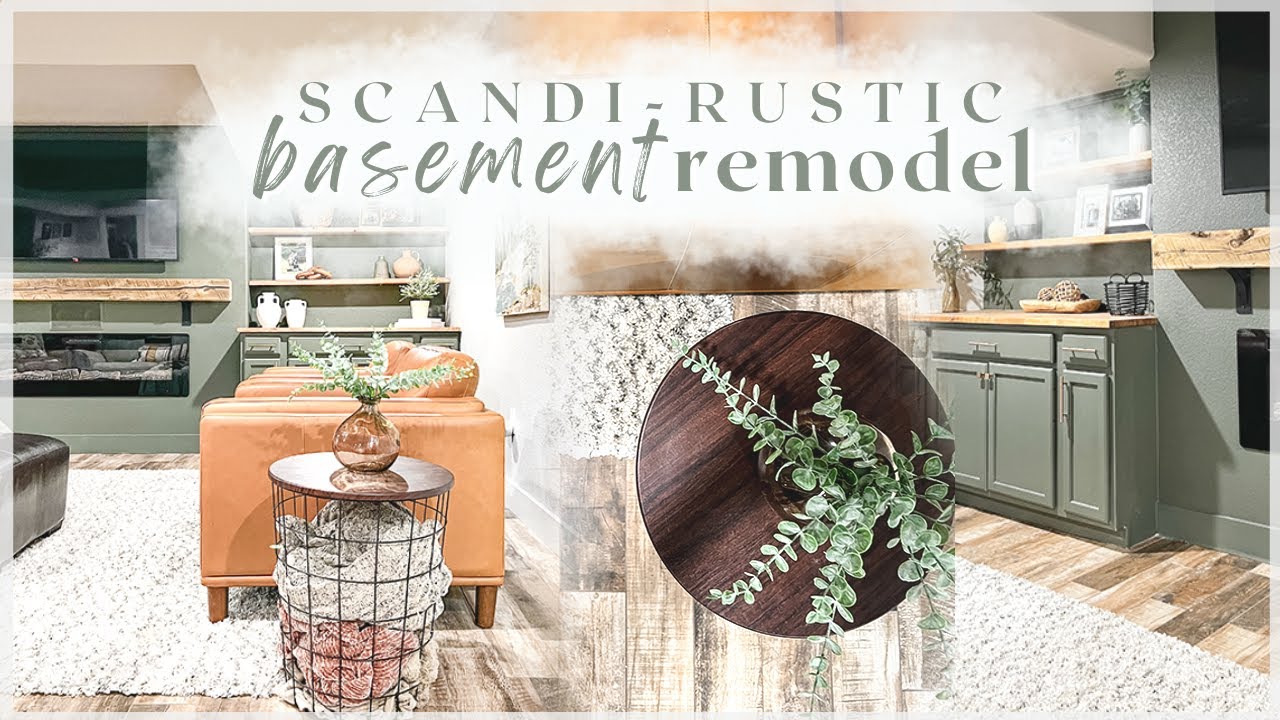The graphic image titled "Scandi Rustic Basement Remodel" features a detailed depiction of a tastefully remodeled basement with Scandinavian rustic design elements. The left section of the photo showcases a cozy living area featuring an olive green wall adorned with inset shelving, holding various decorative items. Below a small wooden mantle, there is a compact fireplace topped by a mounted TV. A light tan leather couch is paired with a black ottoman, creating a comfortable seating area. Nearby, a unique side table made from a wired case with an open design is topped with a wooden platform and a green plant. Single brown chairs are positioned beside the side table on light brown wood floors, partially covered by a white rug. 

The central part of the image provides a bird's eye view of the side table, emphasizing the wooden surface and the green plant. To the right, a close-up reveals more details of the surrounding cabinetry and shelving on the opposite side of the TV. The cabinetry, in matching olive green, features drawers and a wooden countertop adorned with plants, vases, pine cones, and a basket. The harmonious blend of wood and green tones, along with the strategic placement of decorations and furniture, creates an inviting and stylish basement space that embodies the Scandi Rustic aesthetic.